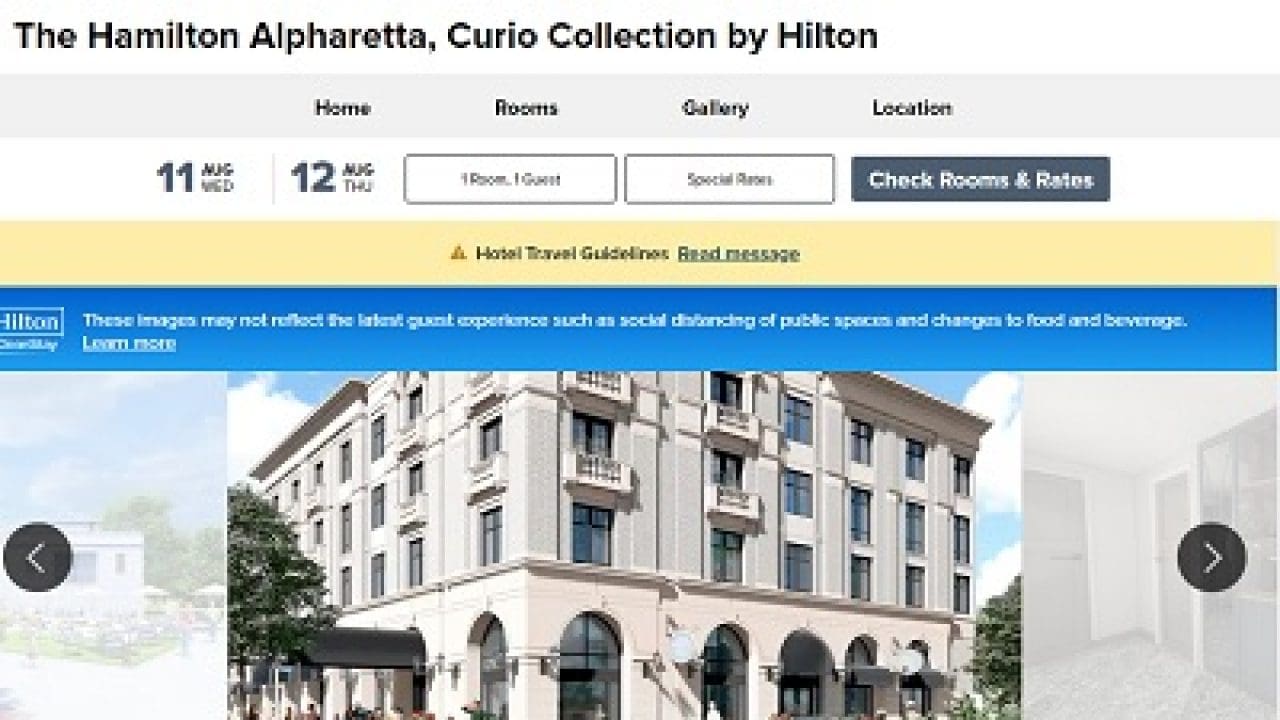The screenshot depicts the official website of the Hamilton Alpharetta, a hotel that is part of the Curio Collection by Hilton. At the top of the page, the hotel's name is prominently displayed. Below this, a navigation bar in a gray horizontal rectangular box with black text lists the categories: Home, Rooms, Gallery, and Location.

Directly beneath the navigation bar, the image displays selected dates: Wednesday, August 11th, and Thursday, August 12th. To the right of the date selection are two white rectangular buttons with black text. The first button denotes “One Room, One Guest,” while the second button is labeled “Special Room.” To the far right, a third dark blue button with white text reads “Check Rooms and Rates,” which is highlighted indicating it is ready for interaction.

A yellow rectangular banner follows, displaying a notice about "Hotel Travel Guidelines," accompanied by a link to "Read Message."

Under this banner, the image features a photograph of the hotel itself. Above the photograph, a disclaimer note says, "These images may not reflect the latest..." (the rest is illegible), and in the upper left corner, "Hilton" is written in white text. The visible portion of the building is four stories tall, featuring a light beige exterior with arches on the ground level. A black awning covers one of the entrances, and several of the rooms have visible balconies.